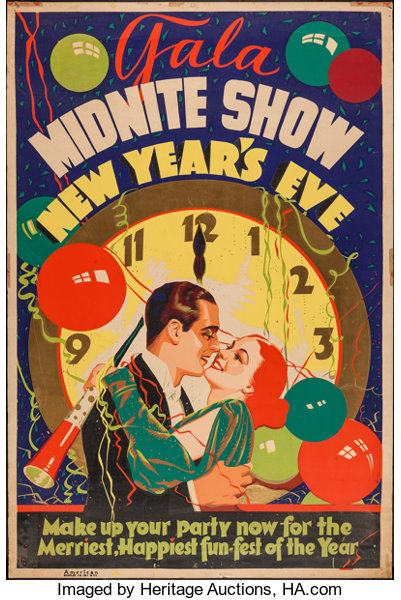This vibrant vintage poster, likely from the 1940s or 1950s, advertises a gala midnight show for New Year's Eve. A circular clock dominates the upper portion of the image, its hands pointing to midnight, symbolizing the start of the New Year. The clock features a brown outer rim and a yellow face, encircled by multicolored balloons—red, teal, green, and blue—that seem to float upward.

Below the clock, a romantic scene unfolds: a European-descended couple is about to kiss amidst a shower of confetti and streamers. The man, tall, dark, and handsome, is dressed in a black tuxedo with brown hair, and he embraces a woman with bright red hair wearing a teal dress. Both are surrounded by a festive ambiance as they gaze into each other's eyes, ready to welcome the New Year with a kiss.

The poster's background is a rich royal blue with a beige border. The event title, "Gala Midnight Show New Year's Eve," is boldly painted in red at the top. At the bottom, the text reads, "Make up your party now for the merriest, happiest fun fest of the year," set against a dark gray or black background with a red border. The image is credited to Heritage Auctions, HA.com, marking this as an exciting and historical New Year's Eve celebration poster.